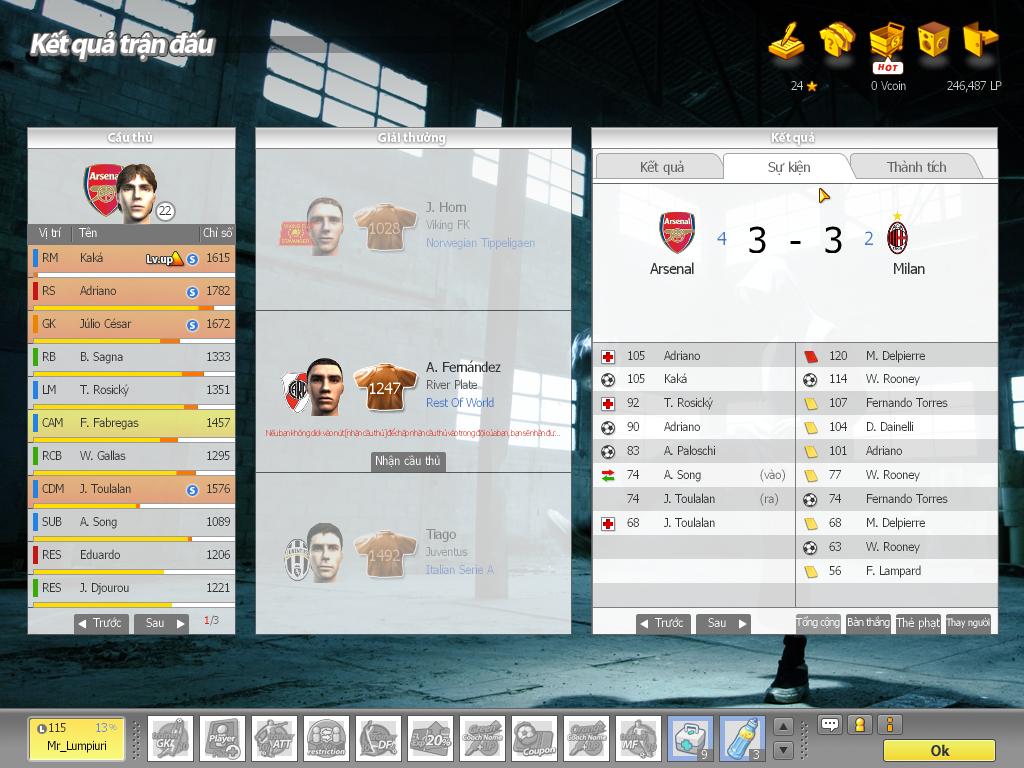The image depicts a football-themed computer game showcasing a match between Arsenal and Milan. Prominently displayed on the screen are the names of various football players, including Ev Fernandes, Thiago, Jay Holm, Adriano, Kala, and Deidre. Notably, Wayne Rooney is listed with identifiers such as number 77 and 114. The background of the image interestingly features a surreal setting that resembles a warehouse with a messy concrete floor, which contrasts with the football-related content. Superimposed on this unconventional backdrop are graphical elements like scoreboards featuring characters’ names and the logos of the Arsenal and Milan teams, adding to the intricate and immersive nature of the game's interface.